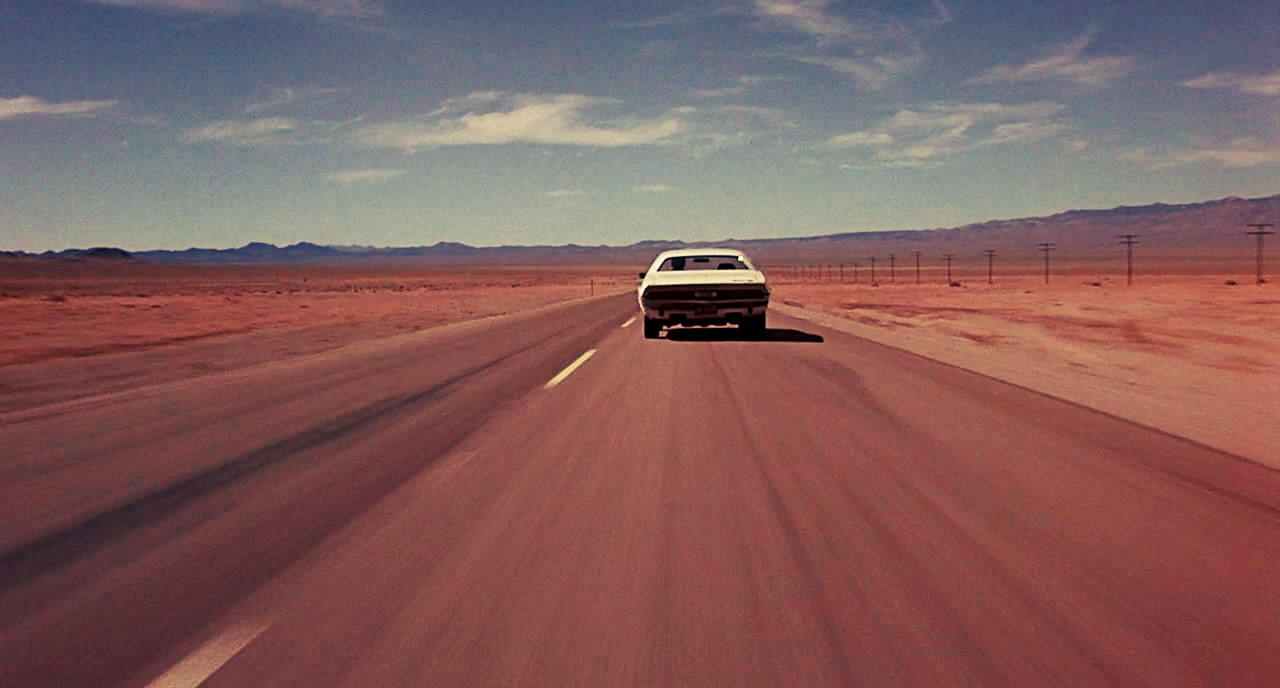In the middle of this image, a solitary vintage white car drives down a deserted two-lane highway, roughly aligned to the right side of the road. The dark gray asphalt with a hint of reddish-brown sand stretches into the distance, bordered by expanses of barren, muddy fields. Far off, a range of rugged mountains creates a rocky horizon. To the right, a series of utility poles punctuates the desolate landscape. Overhead, a brilliant blue sky, painted with wisps of white clouds, arches like a fragile canopy, creating a striking contrast with the earth-toned scenery below. The car—a classic, possibly from the 1960s or 1970s—features a single driver, emblematic of the era's iconic design. The head of the driver is visible, adding a solitary human element to this remote and captivating scene.